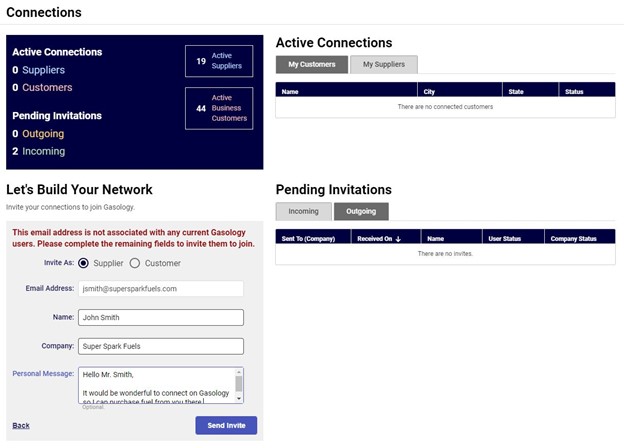In this detailed image of a connection page on the Gasology platform, a variety of sections and messages are displayed:

- The header reads "Connections" with subheaders for "Active Connections" and "Pending Invitations."
- The current status shows "19 active suppliers," "0 suppliers," and "44 active business customers," but indicates "0 customers."
- Under "Pending Invitations," it lists "0 outgoing" but "2 incoming."
- There is a prompt that reads, "Let's build your network. Invite your connections to join Gasology."
- A warning message informs, "This email address is not associated with any current Gasology users. Please complete the remaining fields to invite them to join."
- Fields for inviting connections are presented, including options to "Invite as supplier" or "Invite as customer."
- The email address field contains "jsmith@supersparkfuels.com," with the name "John Smith" and the company "Superspark Fuels."
- The accompanying personal message says, "Hello Mr. Smith, it would be wonderful to connect on Gasology so I can purchase fuel from you there."
- Buttons for "Back" and "Send Invite" are at the bottom of the invitation form.
- The status of "Pending Invitations," "Incoming," "Outgoing," and "Active Connections" is reiterated.
- Subsections such as "My Customers" and "My Suppliers" appear, with columns for "Name," "City," "State," and "Status."
- It clearly states, "There are no connected customers."

The image thoroughly captures the process and details of managing connections and invitations on the Gasology platform.